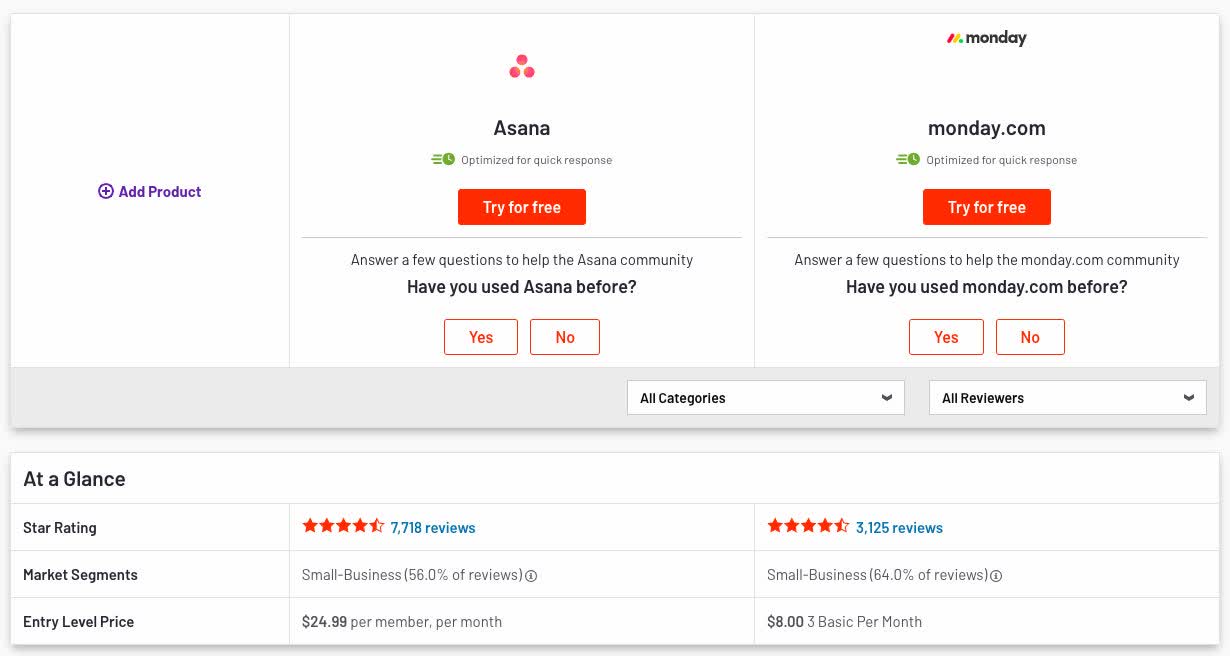This image is a screenshot from an unknown source, likely a comparison website or product review platform. It is divided into two primary sections.

The top section is subdivided into three separate parts:
1. **Add Product**: A simple section represented by a plus sign inside a circle.
2. **Asana**: Featuring an icon of three red dots arranged in a triangular formation, this section promotes Asana with the tagline "Optimize for quick response" and offers a free trial. It prompts the user with the question, "Have you used Asana before?" alongside options for "Yes" and "No." Additionally, it mentions an initiative to gather user feedback with the phrase, "Answer a few questions to help the Asana community."
3. **Monday.com**: Presented in lowercase black letters, this section highlights monday.com with the same tagline, "Optimize for quick response," and offers a free trial. Similar to the Asana segment, it asks, "Have you used monday.com before?" with options for "Yes" and "No." It also mentions a user feedback initiative with the phrase, "Answer a few questions to help the monday.com community."

Below these segments, there is a general filter option described as "All categories, all reviewers."

The bottom section of the image is a long white rectangle providing a detailed comparative overview:
- **Asana**:
  - Star Rating: An average of 4.5 stars based on 7,718 reviews.
  - Market Segment: 56% of reviews from small businesses.
  - Entry-Level Price: $24.99 per member per month.

- **Monday.com**:
  - Star Rating: An average of 4.5 stars from 3,125 reviews.
  - Market Segment: 64% of reviews from small businesses.
  - Entry-Level Price: $8.03 for the basic plan per month.

The image contains no photographic elements, relying solely on text and minimalistic icons for conveying information.